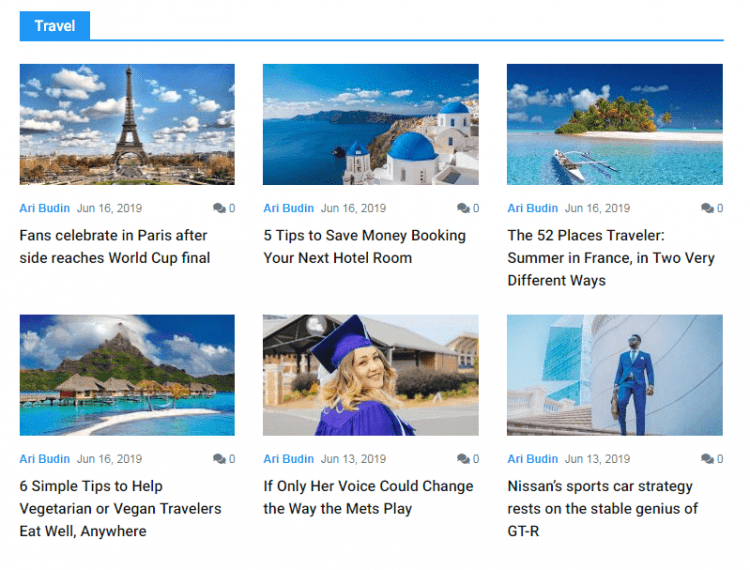The image is a screenshot of a website with a structured layout. At the top of the screenshot, there is a small blue square featuring the word "Travel" in white text with a capital "T." To the right of this word is a thin horizontal line extending across the page.

Below this header area, the content is divided into two rows, each containing three graphical elements or articles. 

Top Row:
1. The first graphic in the top row presents an image of Paris with the Eiffel Tower, accompanied by the headline: "Fans celebrate in Paris after side reaches World Cup final." The name "Arriboudin" is displayed above this caption.
2. The second graphic showcases an image reminiscent of Greece, titled: "Five trips to save money booking your next hotel room."
3. The third graphic depicts an island and carries the text: "The 52 Places Traveler - Summer in France in Two Very Different Ways."

Bottom Row:
1. The first graphic in the bottom row is titled: "Six Simple Tips to Help Vegetarian or Vegan Travelers Eat Well Anywhere." The text is displayed with a focus on providing travel tips for dietary preferences.
2. The second graphic shows a graduate and features the caption: "If Only Her Voice Could Change the Way the Mets Play."
3. The third graphic portrays a person sitting in front of an office building with the caption: "Nissan Sports Car Strategy Rests on the Stable Genius of GT-R."

This overall structure provides a visually organized layout for travel-related content, integrating images and headlines to attract the reader's attention.